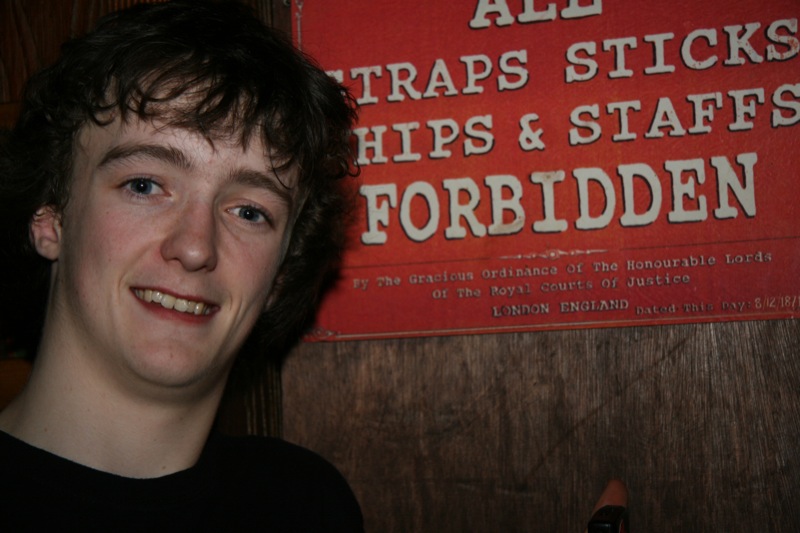In this photograph, a young man, possibly in his late teens to early 20s, is taking a close-up selfie. His head, neck, and part of his shoulders dominate the image, and he is smiling, showcasing his green eyes and dark brown curly hair. He wears a dark shirt and stands in front of a textured wooden wall. Behind him is an orangish-red sign with white text that reads, "All straps, sticks, chips, and staffs forbidden. By the gracious ordinance of the Honorable Lords of the Royal Courts of Justice, London, England," with some smaller, indecipherable fine print below. The lighting on him is poor, suggesting it might have been taken with a flash. Overall, the setting and the sign hint at a historical or official backdrop, possibly in London, England.